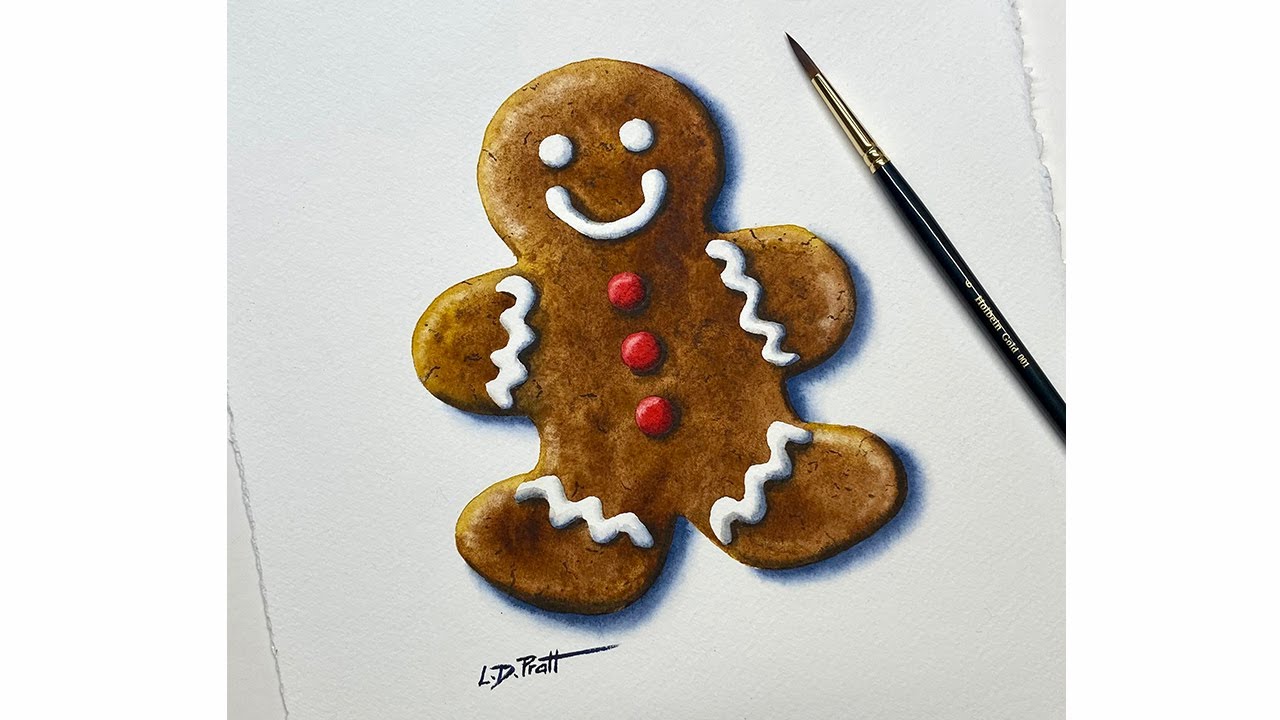The image features a detailed painting of a gingerbread man cookie on a slightly torn white canvas. The gingerbread man is depicted in a rich brown color and adorned with white icing that forms squiggly lines on its stubby arms and feet. It has two white, beady eyes made of frosting, and a large, cheerful smile also in white icing. The gingerbread man has three red buttons, likely representing cinnamon candies, running down its front. A subtle black drop shadow extends to the right of the gingerbread man, adding depth to the artwork. To the right of the gingerbread man, there is a black paintbrush with a silver-colored top. The artist's signature, "L.D. Pratt," is inscribed in black at the bottom of the gingerbread man's left foot, and nearby, the text "Holbein Gold 001" is also visible, likely indicating the paintbrush used to create the piece.